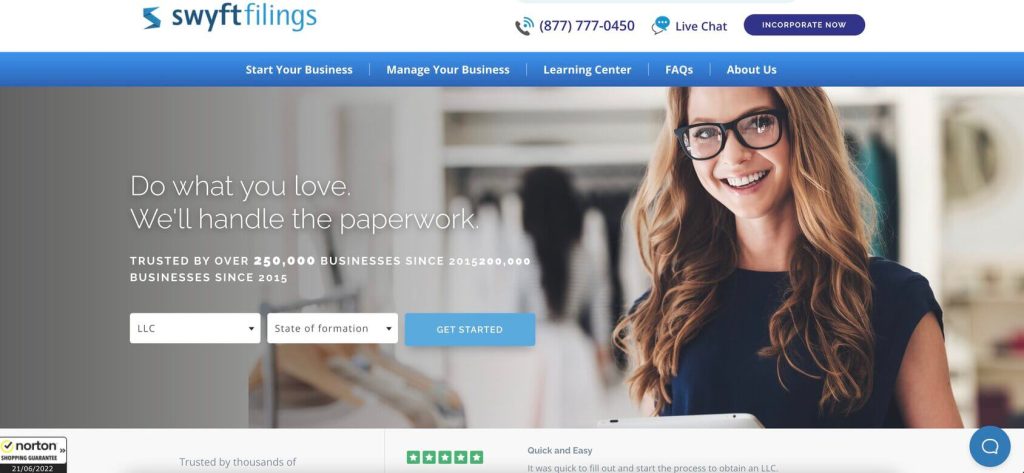The image features a detailed interface layout for a service platform named "Swyft Filings." At the top left corner, there is an emblem resembling an "S" in light blue. Adjacent to the emblem, the words "SWYFT FILINGS" are displayed prominently; "SWYFT" in dark blue and "FILINGS" in light blue. A light blue line runs across the top of the image.

Below the heading, there are several icons and features presented in a structured manner. On the left, there's an icon of a telephone accompanied by a Wi-Fi signal symbol, next to it is a telephone number. Adjacent to this, there are two speech bubble icons, one outlined in grey and the other filled with blue, with the label "Live Chat."

Further down, there is a purple rectangle with bulging sides containing some text, and beneath it is a blue rectangle with the phrase "Start Your Business."

Following this section, a horizontal menu includes options such as "Manage Your Business," "Learning Center," "FAQs," and "About Us," each separated by white lines. 

Below the menu, there's an image of a woman with glasses and long light brown hair situated in what appears to be a clothing shop. The left side of the image is predominantly grey, shifting to more vivid colors towards the right. Overlaid text reads "Do what you love, we'll handle the paperwork." Additional text in white is displayed beneath this tagline.

Directly below the image are interactive elements, including white rectangles marked "LLC" and "State of Formation," both featuring dropdown arrows. There is also a blue rectangular button labeled "Get Started."

At the bottom of the image, there's a black-outlined rectangle containing a yellow checkmark with the text "Norton Secured." Below this are some additional words. The footer features a black rectangle with grey text, followed by a row of five green squares each containing a white star. Finally, there is a blue circle with a white outlined speech bubble within it.